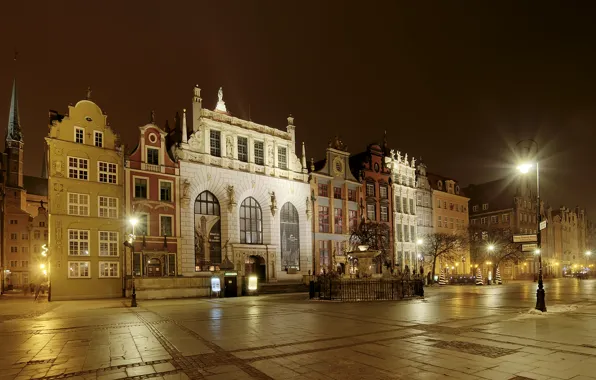This nighttime photograph captures a charming and ornate street scene in a European city. The scene is illuminated by tall black street lamps, casting a gentle glow on the smooth surface of a white brick sidewalk that extends between eight distinct buildings. Each building varies in height and style: the tallest one, centrally located, boasts five stories and is finished in elegant white brick with arched windows, while others are crafted from green brick, red brick, and other materials, creating a visually captivating array of architectural designs. This courtyard-like area features a stone and brick street with a prominent fountain or wishing well situated in the center, drawing people's attention as they gather around it. The ambiance is further enhanced by the presence of trees in the distance, making it a picturesque urban block a mix of residential and possibly downtown elements.